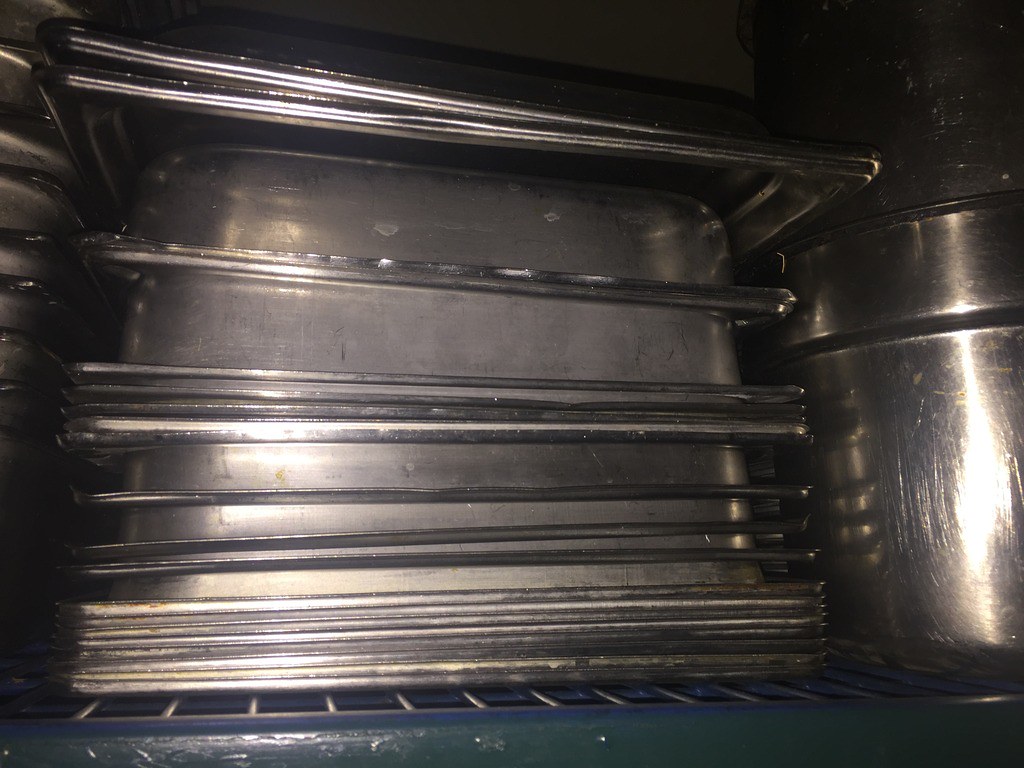This detailed photograph captures a close-up of a high-quality, heavy-duty steel grate rack in an industrial kitchen, displaying a meticulously organized stack of reflective stainless steel pans. The pans, varying in height and size, are neatly arranged with the smallest and thinner pans forming the base, progressing upward to larger, deeper pans. Some of these deeper pans are designed to fit into steamer tables commonly used in buffet-style setups. At the very top of the stack, a couple of cookie sheets rest, completing the arrangement. To the right of this stack stands a large stainless steel pot, roughly the same height as the stack itself. The overall scene is slightly obscured by low lighting, with a dark background that adds a degree of ambience but makes the details a bit challenging to discern. The cleanliness and order suggest that these kitchen tools have been prepared and are ready for their next use.